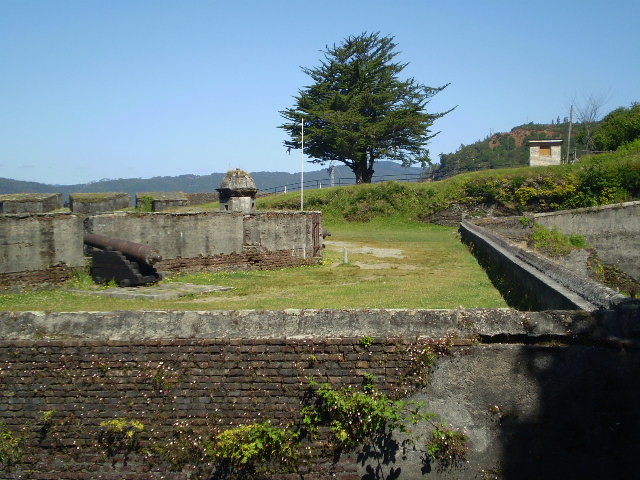The image captures an outdoor setting bathed in daylight with a clear blue sky. A very old and worn stone and brick wall dominates the foreground, structured in a zigzag pattern. At the base of this wall, a few branches with leaves are visible. This primary wall encloses a central courtyard. Toward the middle right, there is a large metal object, likely an aged cannon, perched atop a concrete structure resembling a staircase. This structure has a turret-like area with a flagpole. The courtyard features patches of grass mixed with dirt, surrounded by more concrete formations and another old stone wall to the left. In the distance, a tall tree stands against the backdrop of the blue sky, framed by mountains and a small square shed-like structure on the right. Sparse greenery, including grass and shrubbery, is scattered around the concrete structures, enhancing the historical and slightly rundown ambiance of the scene.